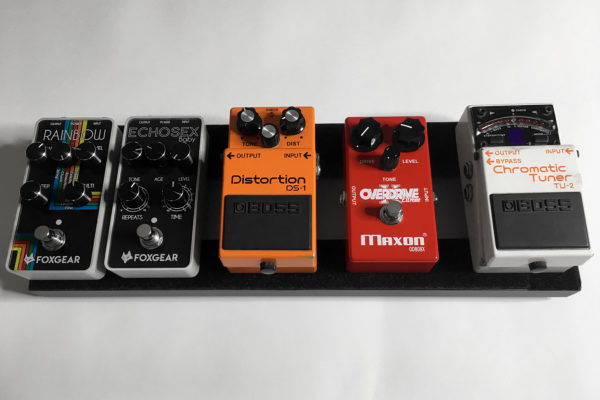The image depicts a collection of five guitar pedals arranged on a black rectangular stand, all centered against a white background. From left to right, the first two pedals are black and branded as Foxgear. The leftmost pedal features rainbow stripes and is labeled "Rainbow," while the second pedal is labeled "Echosex." Each of these two pedals has six dials—five black and one silver, with the silver likely being a button. The third pedal in the center is an orange distortion pedal labeled "Distortion DS-1," with three black dials. The fourth pedal is a red overdrive pedal marked "Overdrive 2," branded as Maxon, and it also has three black dials. The final pedal on the right is a white chromatic tuner labeled "Chromatic Tuner TU-2" with red text, branded as Boss. The chromatic tuner features input and output labels, along with a scale with red text numbers at the top. The overall setting appears to be a home or recording studio.